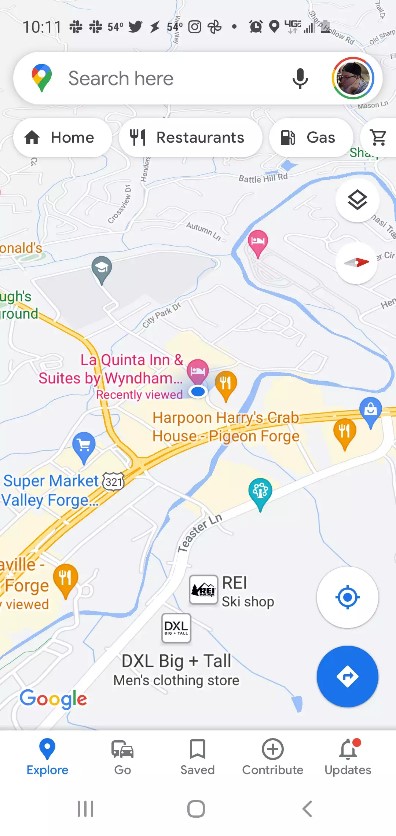The screenshot on the Android phone displays the Google Maps app, pinpointing the user's precise location with a prominent blue dot. The map showcases the immediate vicinity, prominently featuring the La Quinta Inn & Suites by Wyndham at either Valley Forge or Pigeon Forge, as indicated by the names of surrounding restaurants, supermarkets, and other landmarks. At the top of the screen, below the search bar, are typical Google Maps menu options, including shortcuts to search for home, restaurants, and gas stations. At the bottom, another menu bar offers buttons such as Explore, Go, Save, Contribute, and Updates for navigation and location management. The user's profile picture in the top right corner confirms that they are logged into their Google account.